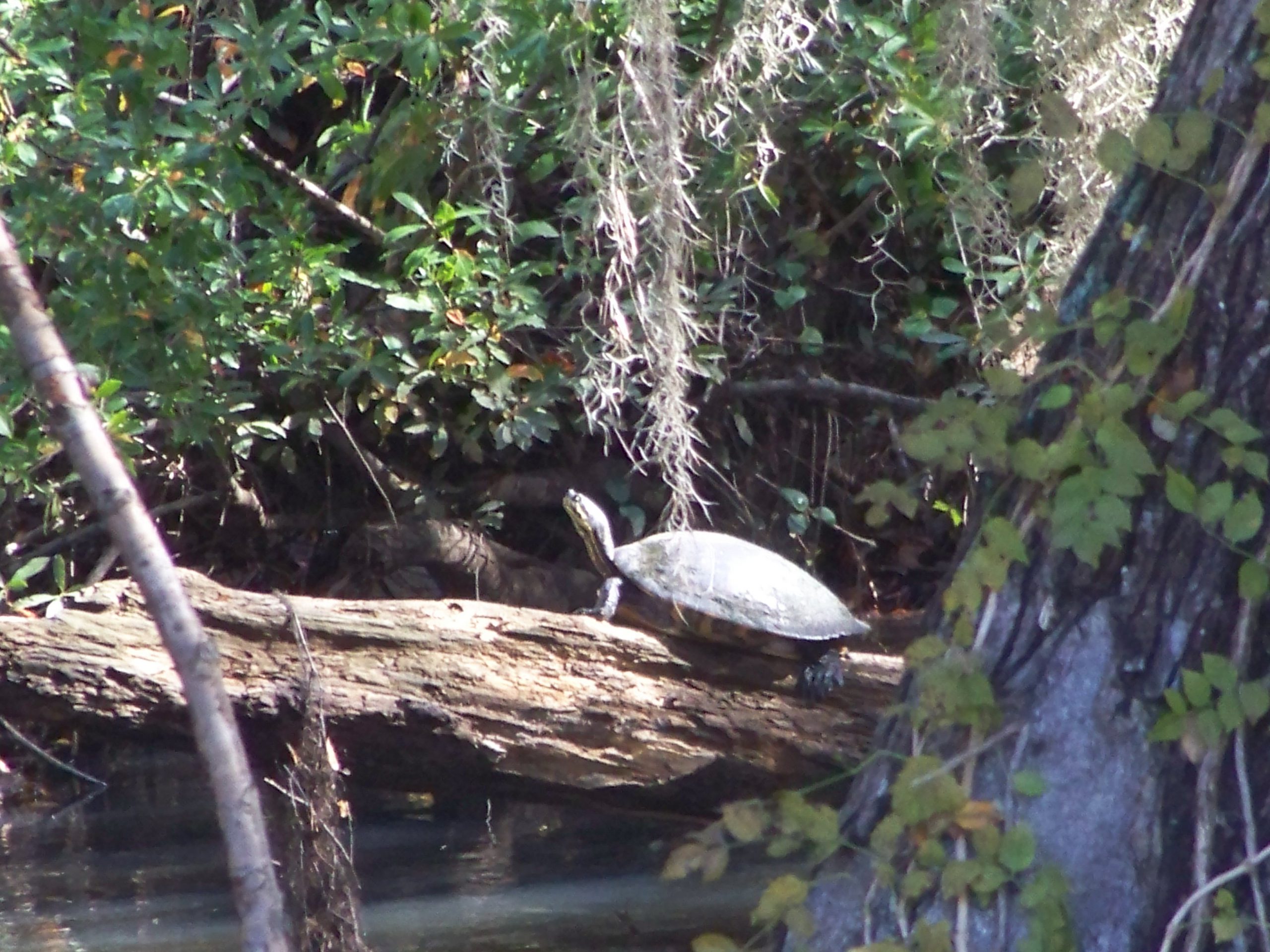This outdoor photograph captures a serene nature scene in a horizontal landscape orientation. At the center, a turtle basks in the sunlight on a decaying branch that spans over dark blue water, likely a lake or river. The turtle is oriented with its head facing the upper left corner and its neck slightly extended, enjoying the warmth of the sun, which reflects off its shell and head. Surrounding the turtle, greenery abounds: there are branches with green leaves overhead, and some white hanging moss drapes down near the turtle. To the right, a thicker tree trunk adorned with vine-like leaves stands partly in shadow. The image does not reveal the sky directly but suggests bright conditions above, emphasizing the reflective light off the turtle and water.